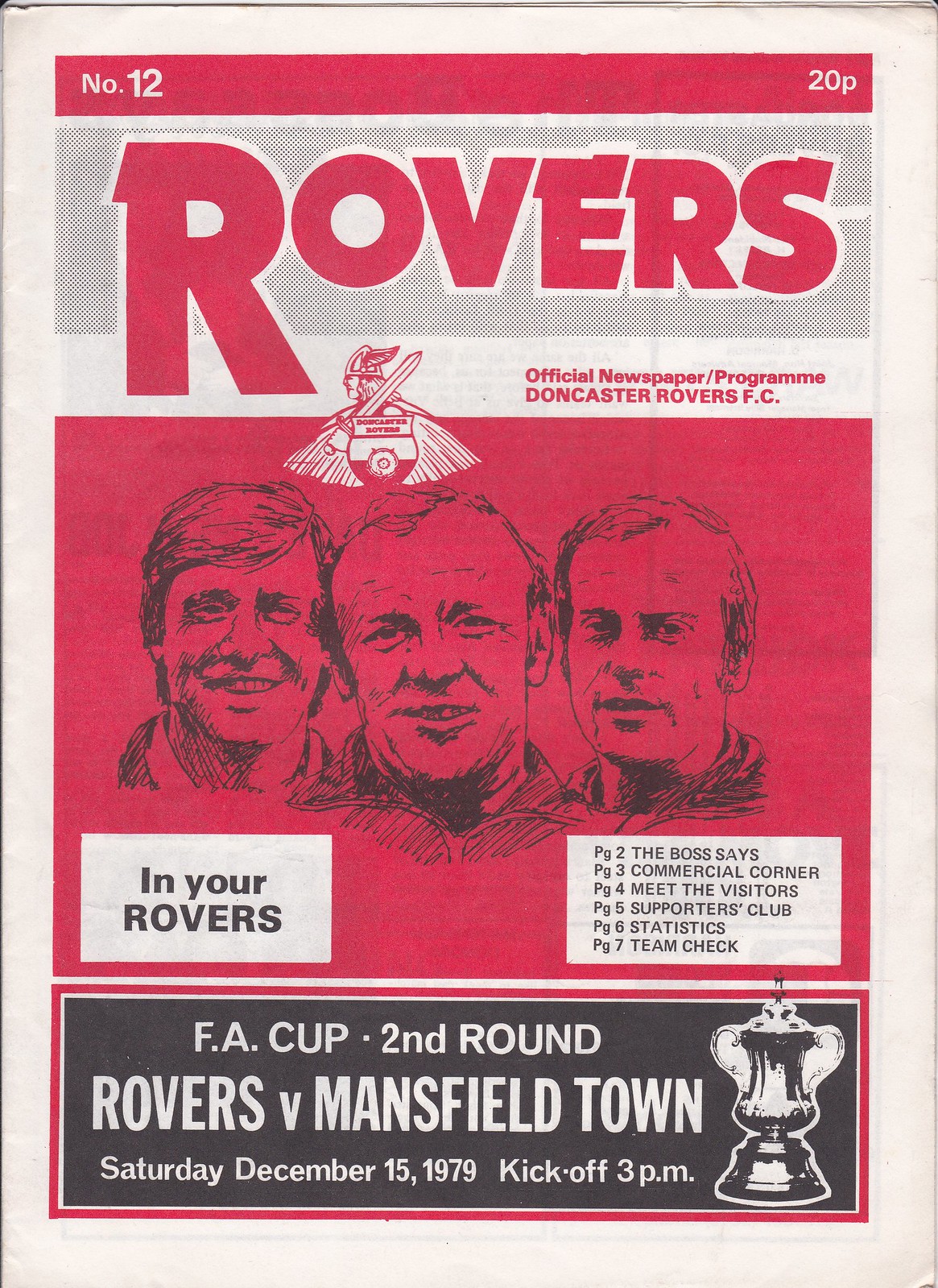The image is of a vintage magazine cover for the official newspaper and program of Doncaster Rovers FC, styled predominantly in red, white, and black. At the top, a red bar with white text details "No. 12" on the left and "20p" on the right. Below this, a grey box prominently features the title "ROVERS" in large, bold red letters. Beneath the title, the text "official newspaper/program Doncaster Rovers FC" appears in red on a white background. Central to the cover is the club emblem, depicting a Viking holding a sword, situated above a black and white artist's sketch of three men's faces. The sketch occupies a red background and shows the men smiling. Below this illustration, a series of white boxes with black text lists contents: "Page 2: The Boss says, Page 3: Commercial Corner, Page 4: Meet the Visitors, Page 5: Supporters Club, Page 6: Statistics, Page 7: Team Check." The bottom of the cover features a black box with a red border, containing white text that announces "FA Cup Second Round, Rovers vs. Mansfield Town, Saturday, December 15, 1979, Kickoff 3 p.m." To the right within this black box is a small black trophy illustration. The entire cover rests on a cream-colored background, suggesting the aged and nostalgic quality of the magazine.